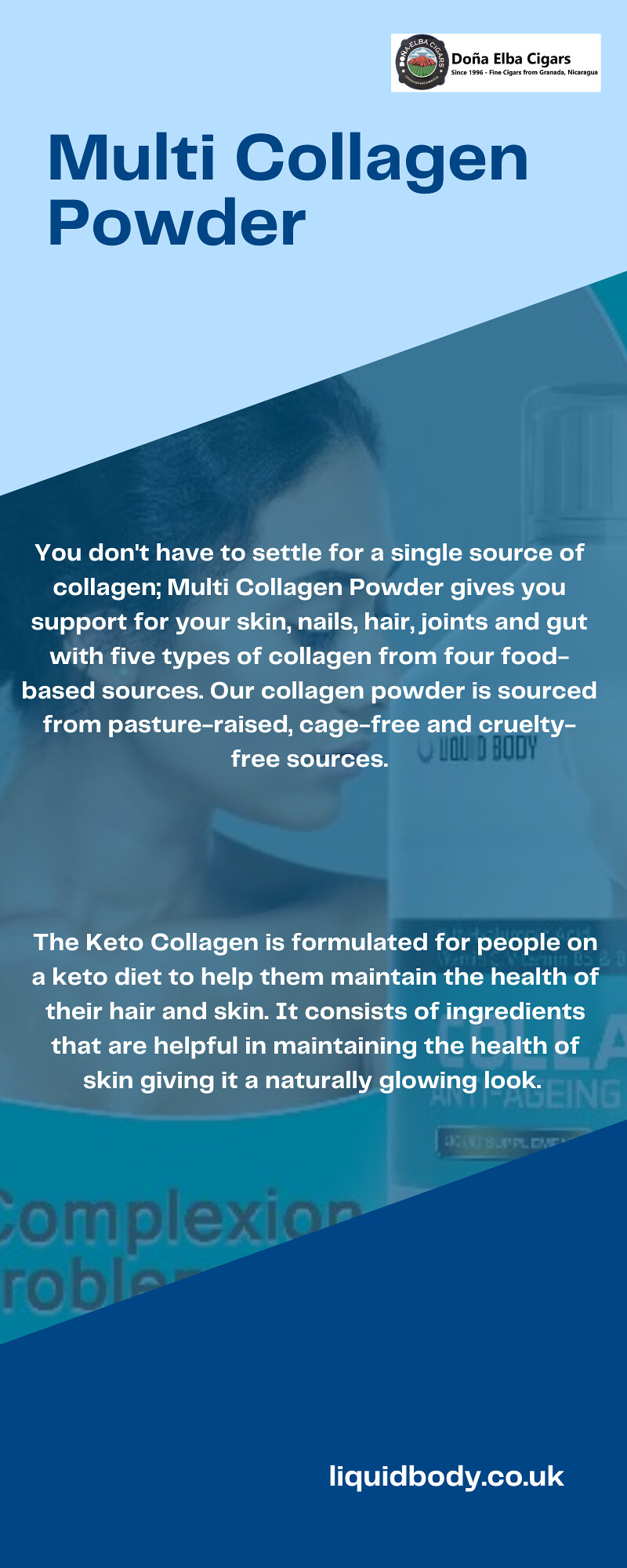This detailed, colorful advertisement for Liquid Body’s multi-collagen powder showcases a gradient of three shades of blue: light blue at the top, middle blue in the center, and dark blue at the bottom. The top prominently features the title "Multi-Collagen Powder," while the bottom displays the website "liquidbody.co.uk." Sandwiched between these sections are two informative paragraphs. The first highlights the benefits of the multi-collagen powder, emphasizing its support for skin, nails, hair, joints, and gut health through five types of collagen derived from four distinct food-based sources. Sourced responsibly from pasture-raised, cage-free, and cruelty-free origins, this powder caters to the health-conscious consumer. The second paragraph focuses on the keto-friendly formulation, specifically designed for those on a ketogenic diet, ensuring the maintenance of healthy, naturally glowing skin. An additional visual element in the background appears to show a woman opening collagen packaging, further enhancing the advert’s appeal.